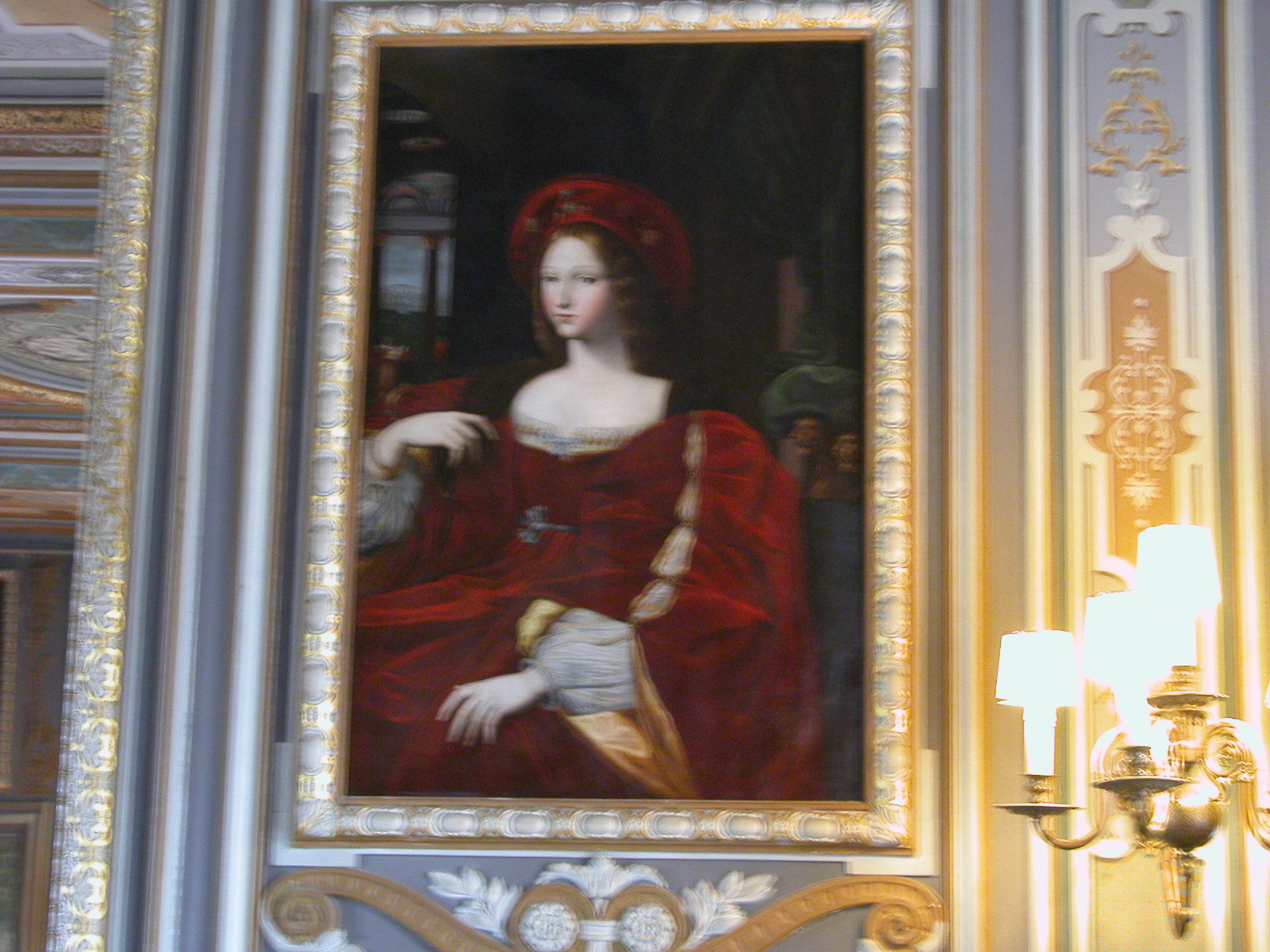The image depicts a blurry photograph of a framed painting mounted on a wall with an intriguing, somewhat metallic bluish tint. The wall is adorned with ornate decorations, including gold fleur-de-lis. To the right of the painting, three light bulbs on a chandelier can be seen, though the fixture appears cut-off. The ornate frame encasing the painting features shades of pale blue, grays, and whites, giving it a shiny and bold appearance, reminiscent of the walls. 

The painting itself showcases an exquisitely detailed portrait of a woman with a Mona Lisa-like facial expression, but distinctly not the famed Mona Lisa. She has dark reddish-brown hair adorned with a large red hat or tam that matches her poofy, long red dress. The background of the painting is dark, with faint hints of additional figures and possibly a window, suggesting an interior setting from a historical era, such as the Middle Ages, Victorian, or Renaissance period. The skilled artistry of the painting stands out, conveying lifelike qualities. The slightly blurred photograph suggests that it was captured in motion, perhaps in a museum or a richly decorated home.